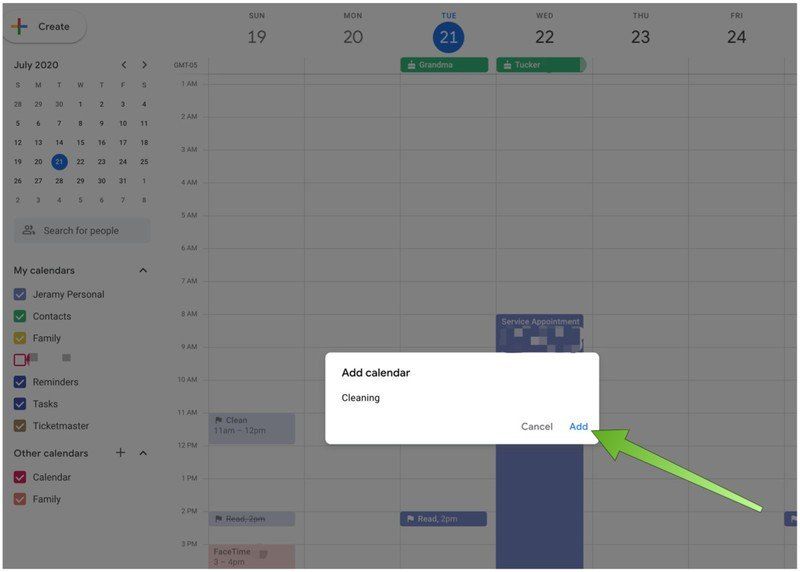This image displays a screenshot of a digital calendar interface from July 2020. In the foreground, near the bottom and center, there is a prominent white box with bold text saying "Add Calendar." Below this heading, it reads "Cleaning." To the right of this text, there are two buttons: one labelled "Cancel" and the other labelled "Add." 

A green arrow ascends from the bottom right corner of the image, pointing directly at the "Add Calendar" section and the specified "Cleaning" calendar. The background calendar shows dates ranging from June 28th to August 8th. Across the top, the highlighted dates include the 19th, 20th, 21st, 22nd, 23rd, and 24th of July, which are part of the current week's view in the calendar grid.

On the left side of the interface, you see a vertical list of numerical dates corresponding to the days within the calendar month. Below this date range, there is a search bar labelled "Search for people," followed by a section titled "My Calendars." The overall design and layout are indicative of typical digital calendar applications, facilitating the organization and scheduling of tasks and events.